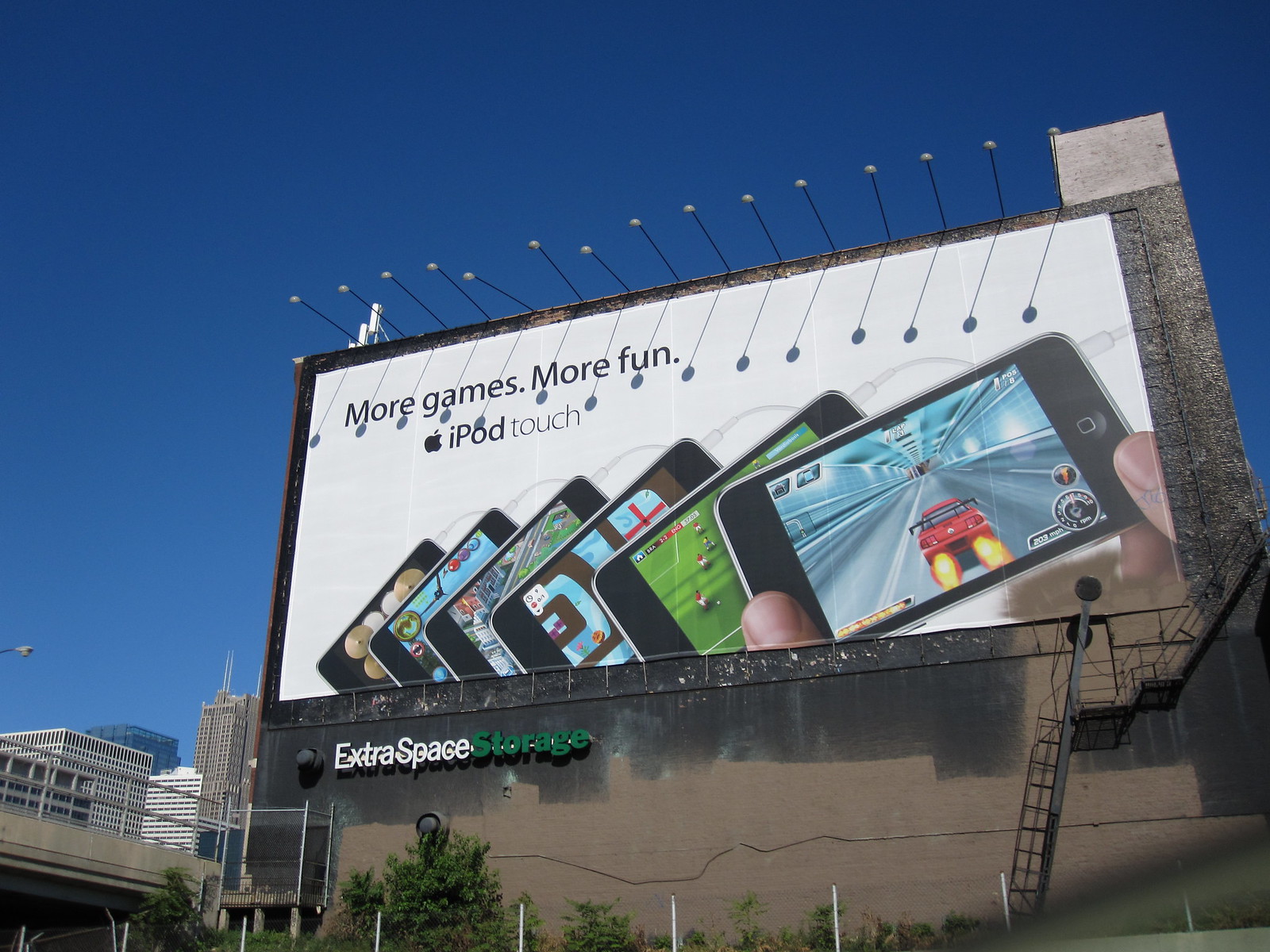The image depicts a large billboard mounted on the gray stone facade of a building in a bustling metropolitan area, under a bright blue sky. The billboard advertises an iPod touch with the slogan “More games. More fun.” in black text on a white background, accompanied by an Apple icon and the words “iPod touch.” Below the slogan, six iPod touches are displayed at various angles, each showing different games on their screens. The left side of the billboard has the words “extra space storage,” with “extra space” in white and “storage” in green, suggesting that the building might be a storage facility. A prominent crack runs through the lower part of the building. On the right side of the structure, there's a set of stairs that lead to a platform below the billboard, accessed by a ladder. Protruding from the top of the building are several poles with reflective circular ends, casting shadows on the billboard below. Adjacent to the billboard, tall city buildings and a construction overpass are visible, enhancing the urban setting of the scene.